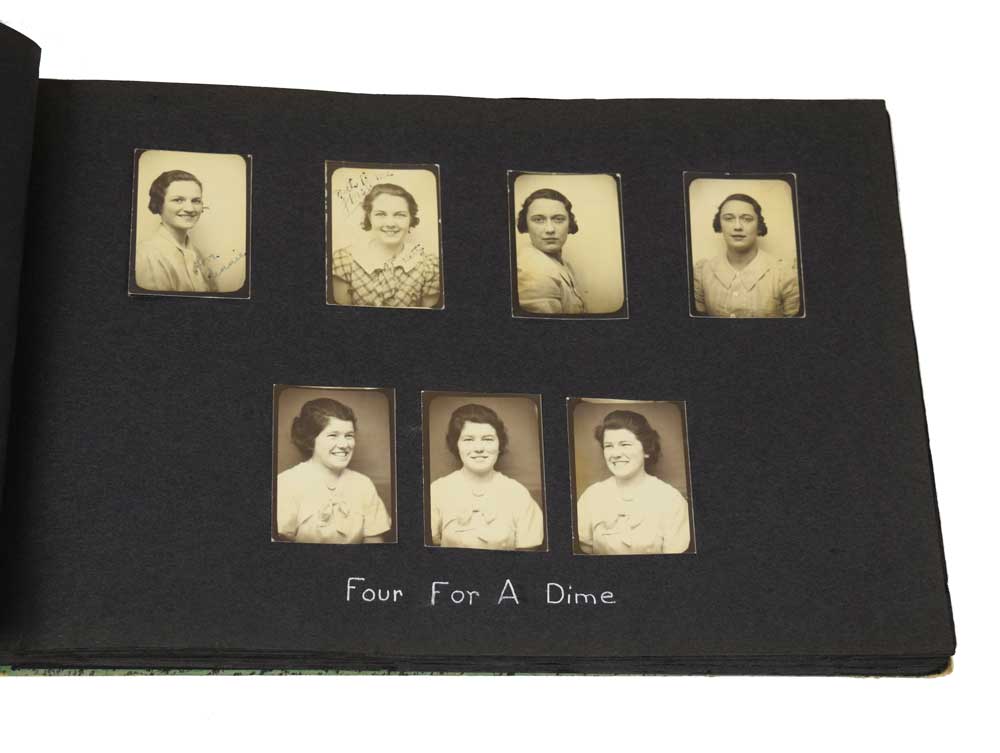This image showcases a page from an antique photo album, featuring a total of seven black-and-white headshots of women. The layout includes four images on the top row and three on the bottom. Each of these headshots presents a woman gazing into the camera, all of whom have short brown hair and are dressed in attire visible from the chest up. Notably, the top row seems to depict three different women, with two instances of one woman's image being repeated, while the bottom row displays three images that might be the same woman shown from different angles, possibly offering side profiles and a centered view. Adding to the historic charm of this collection, a line of text beneath the photos reads "Four for a dime," implying a nostalgic pricing for these portraits. The album itself has a black background, emphasizing the timeless quality of these carefully preserved photographs.